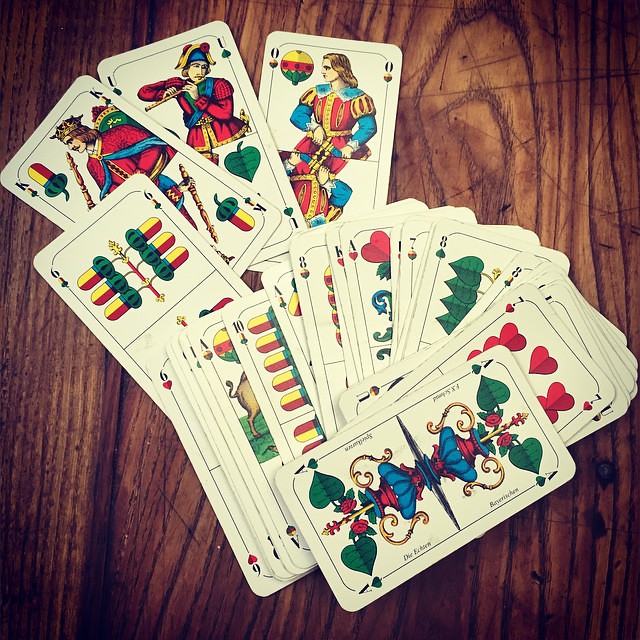The image showcases an array of vintage playing cards meticulously spread out across a rustic wooden table, creating a perfectly square composition. The cards, characterized by their old-fashioned design, deviate from the standard modern deck. Among the visible cards are a king, jack, queen, sevens, eights, an ace, a ten, and a six, alongside partially shown cards, including more aces and another king.

The cards boast a straightforward color palette featuring blue, red, yellow, green, and black, reinforcing their antique aesthetic, which hints at an 18th or possibly 19th-century origin. The dimensions of the cards appear slightly larger than contemporary playing cards, adding to their distinct charm.

A notable detail is the presence of German text on one of the cards, which reads "Bayernschlein," commonly interpreted as "Bavarian little one," as well as “Eichhörn,” meaning “squirrel.” The design is framed by elegant borders, with clear symbols denoting each card's suit and rank, adding to the historical and artistic value of the collection.